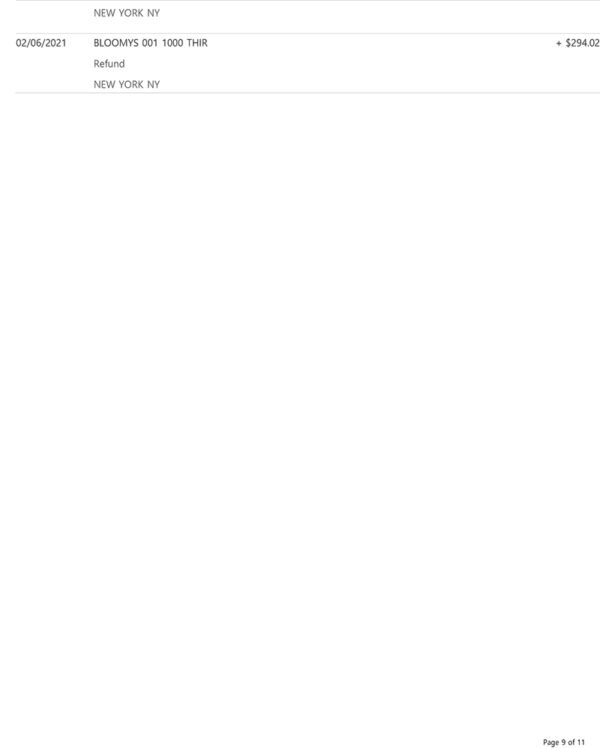This image depicts a digital interface, likely viewed on a computer or a phone screen. At the top left corner, there are three faint gray lines. Immediately below these lines, the text "New York NY" appears in gray font and in all capital letters. On the far left, there is a date displayed as "02/06/2021". Next to the date, there's the label "Bloomys," followed by the sequence "001 1000 THIR", with "THIR" also in capital letters. Directly below this, the word "refund" is visible. Underneath "refund," the text "New York NY" is repeated in all capital letters. A faint gray line delineates this section from the blank space below. Towards the right side of this blank area, there is another section that prominently displays "+$294.02."